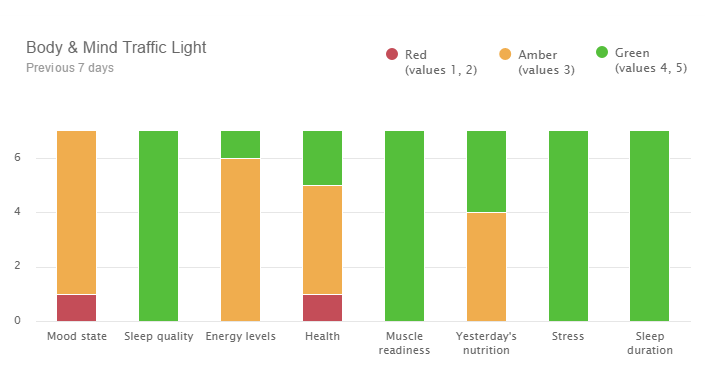The image is a detailed color bar graph titled "Body and Mind Traffic Light" located in the upper left corner in gray text. It displays eight vertical bars that represent various aspects of an individual's life over the previous seven days, including Mood State, Sleep Quality, Energy Levels, Health, Muscle Readiness, Yesterday's Nutrition, Stress, and Sleep Duration. Each bar is color-coded in accordance with a key situated in the upper right corner, illustrating red, yellow, and green segments identified by corresponding dots.

Below each bar are labels in gray text, specifying the different categories tracked. On the left, a numerical scale ascends from 0 at the bottom to 2, 4, and 6, with horizontal gray lines marking each number. The colors of the bars reflect changes in levels: red denotes lower values, amber indicates intermediate values, and green signifies higher values.

The specifically noted trends are:
- Mood State starts in red between 0 and 1, turning amber afterward.
- Sleep Quality is consistently green.
- Energy Levels transition from amber up to value 6, then turn green.
- Health starts in red at 1, shifts to amber by 5, and reaches green at the top.
- Muscle Readiness remains entirely green.
- Yesterday's Nutrition is evenly split between amber and green.
- Stress and Sleep Duration are both entirely green.

This comprehensive visual summary provides an intricate snapshot of the person's well-being in several key areas, color-coded to easily identify periods of concern or stability.